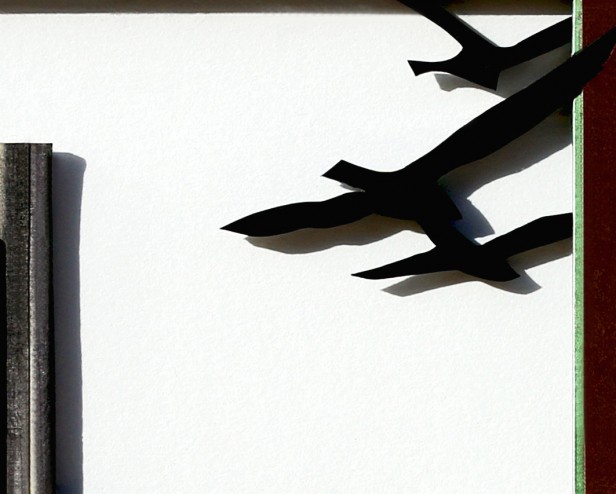This is an abstract, stylized black and white painting, potentially a watercolor, set on a predominantly white background. The image features three black birds with outstretched wings, depicted in an abstract form, flying toward a structure on the left side. The structure, which could be a piling, a dock, or part of a building, is only partially shown and its shadow extends to the right of the frame. The right side of the painting includes a vertical element with a deep wine red color, accented by a small sliver of light blue. Additional details include a thin black border at the top and a subtle green border contrasting against the darker hues of the watercolor. The overall composition is minimalistic yet intriguing, with shadows cast behind the birds and the structure, adding depth and a sense of movement to the otherwise plain, white background.